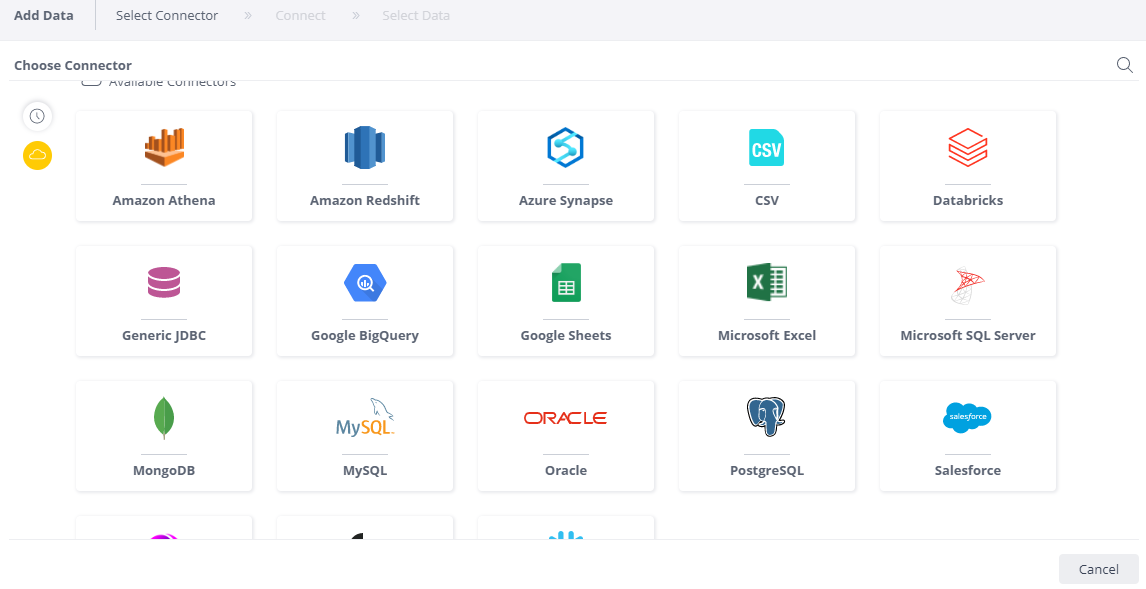The image depicts a detailed web interface chart, framed by a light gray header that is divided into three sections arranged horizontally. The first section on the top left, labeled "Add Data," is marked by bold black text. The subsequent sections are labeled "Select Connector" and "Connect and Select Data," with these latter labels appearing in a grayed-out font. The overall background of the webpage is a clean white, with the title "Choose Connector" prominently displayed in the top left corner.

Below the title, the interface is organized into approximately four rows featuring a total of 18 boxes, each containing an icon and its corresponding label. The layout includes three rows, each with five such boxes. Starting from the left, the first icon represents Amazon Athena and features a vertical bar graph in varying shades of orange. Next to it, the Amazon Redshift icon is depicted by three vertically stacked blue cylinders. The third icon for Azure Synapse is a hexagonal shape with a "Z" in the middle, followed by a teal icon labeled CSV with the letters in white. The Databricks icon has an orange outline and resembles a stack of books.

Additional icons in the interface include:
- Google Sheets
- MySQL
- Oracle
- Microsoft Excel
- Generic JDBC
- MongoDB
- Salesforce
- Microsoft SQL Server

Each section and icon in the chart is crafted to provide a visual and functional understanding of the connectors available for selection, ensuring a comprehensive and user-friendly experience for individuals managing data integration tasks.